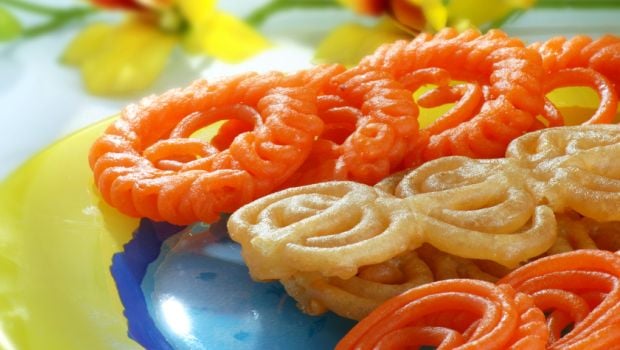The photograph captures a horizontally oriented scene featuring a distinctive collection of food items on an artistic plate. Centered on the plate, which has a blue middle and a yellow rim, are homemade, circular pastries. These light, crispy confections are divided into rows with alternating colors—vibrant orange and a creamy beige. Each pastry is creatively designed with heart-shaped cutouts and made of interwoven dough ropes that indicate their delicate, crumbly texture. The background subtly showcases a stem adorned with yellow flowers resting on a white surface, adding a touch of natural beauty to the setting. The plate itself appears handcrafted, with a dark blue circle and lighter blue accents, enhancing the overall aesthetic charm of the image.